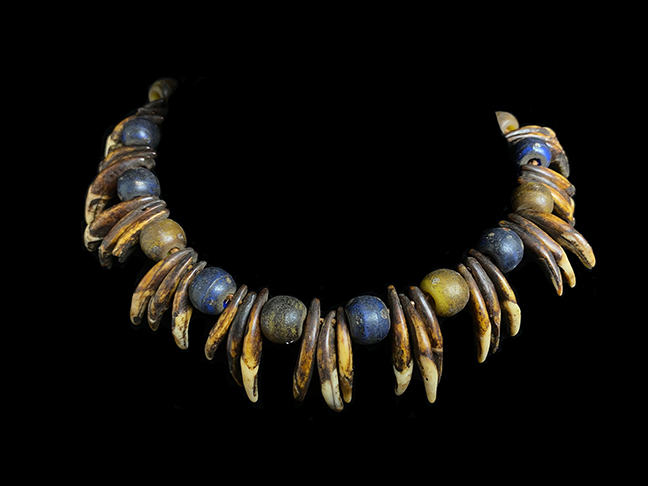The image features an ancient tribal necklace laid against a stark black background. The necklace, adorned with an array of beads and claw-like adornments, seems to float, revealing no visible string or fastening mechanism. Predominantly blue and yellow beads alternate between clusters of similar-looking claws, likely sourced from the same type of bird or animal. The claws are rhythmically interspersed with beads, creating a pattern of three claws followed by a bead. At each end of the open necklace are what appear to be half seashells. There are also green beads sporadically placed within the design. Overall, the piece exudes an ancient, possibly voodoo-like aesthetic, characterized by its tribal craftsmanship and mysterious presence.